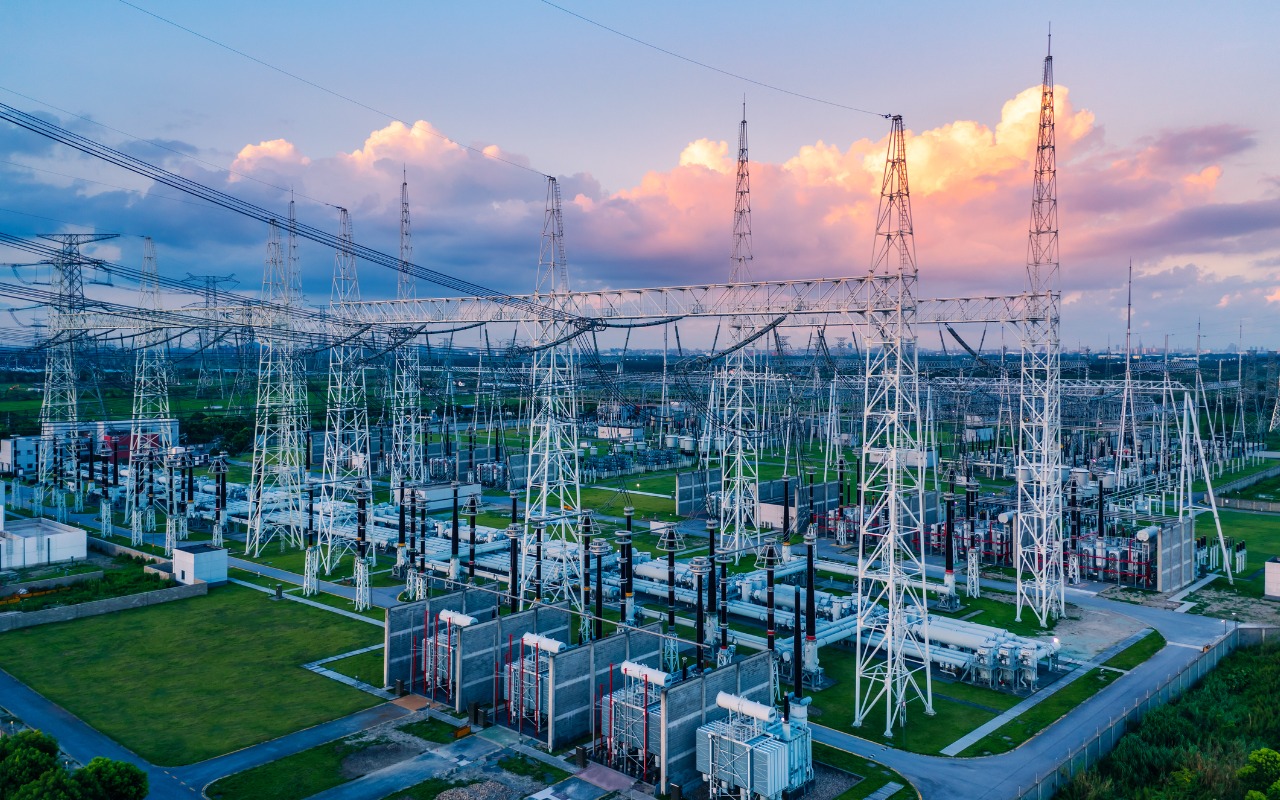The image depicts a vast electrical power plant set against an orange-tinged sunset sky, where thick clouds partially obscure the sun. In the foreground, there are four rectangular blue machines, each topped with a white coil, arranged in a square pattern with concrete walkways and sections of green grass separating them. Moving further into the image, two rows of slim, white metal towers—each connected by a horizontal metal framework—stretch into the distance, flanked by various sets of cables. Taller, thinner black poles are positioned adjacent to many of these white towers. Additionally, white tubes lay along the grassy ground between these two rows of towers. Surrounding the towers are fences and more pathways, with some paths leading off to the right and left, bisecting through patches of lush grass and interspersed shrubs. The intricate network of wires extends out from the tops of the towers, both vertically and diagonally, adding to the complexity of the scene.